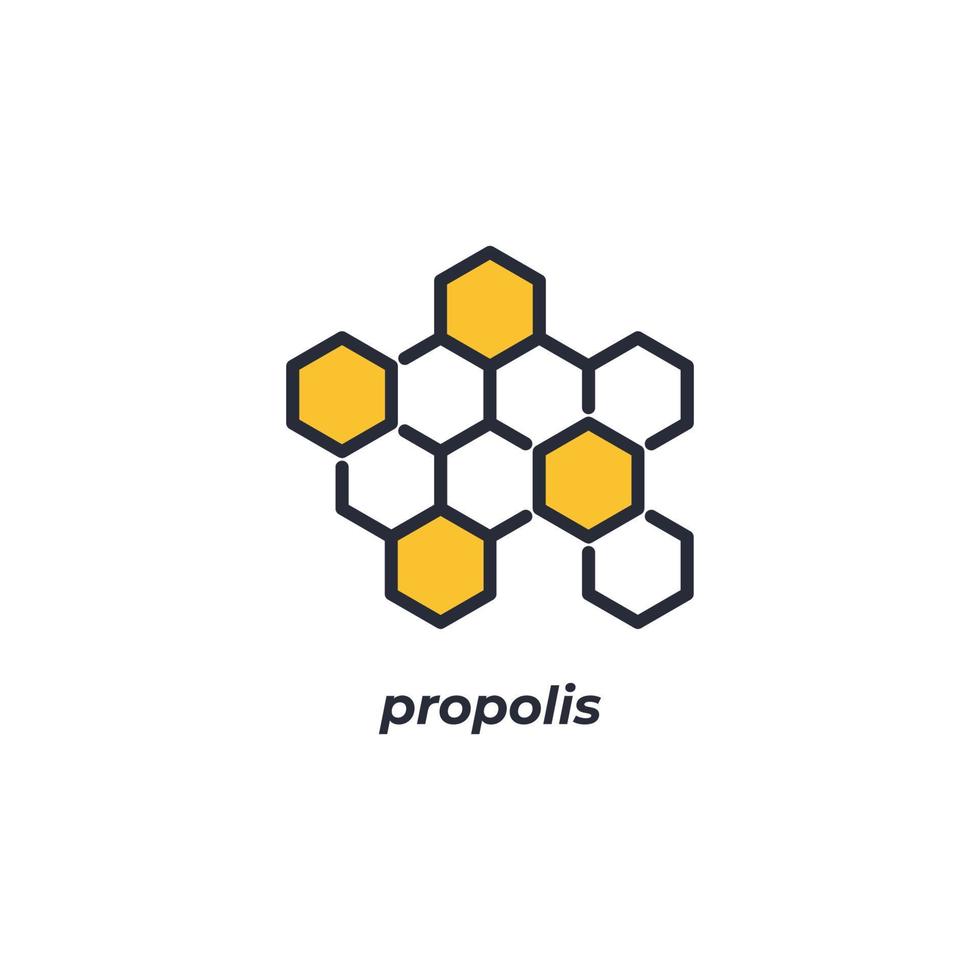The image is a simple logo featuring a honeycomb design against a completely white background. The honeycomb consists of 10 interconnected hexagons outlined in thick black lines. Four of these hexagons are filled with a muted yellow color. The arrangement includes one yellow hexagon at the top center, followed by a horizontal row of four hexagons with the leftmost one being yellow. Beneath this row is a line of three hexagons, with the last one on the right filled with yellow. Finally, there is a yellow hexagon connected to the middle hexagons in the last row. Below this honeycomb pattern, there is the word "propolis" written in black italicized text, all in lowercase letters. The clean and stark design suggests a corporate logo, possibly related to bees or beekeeping.